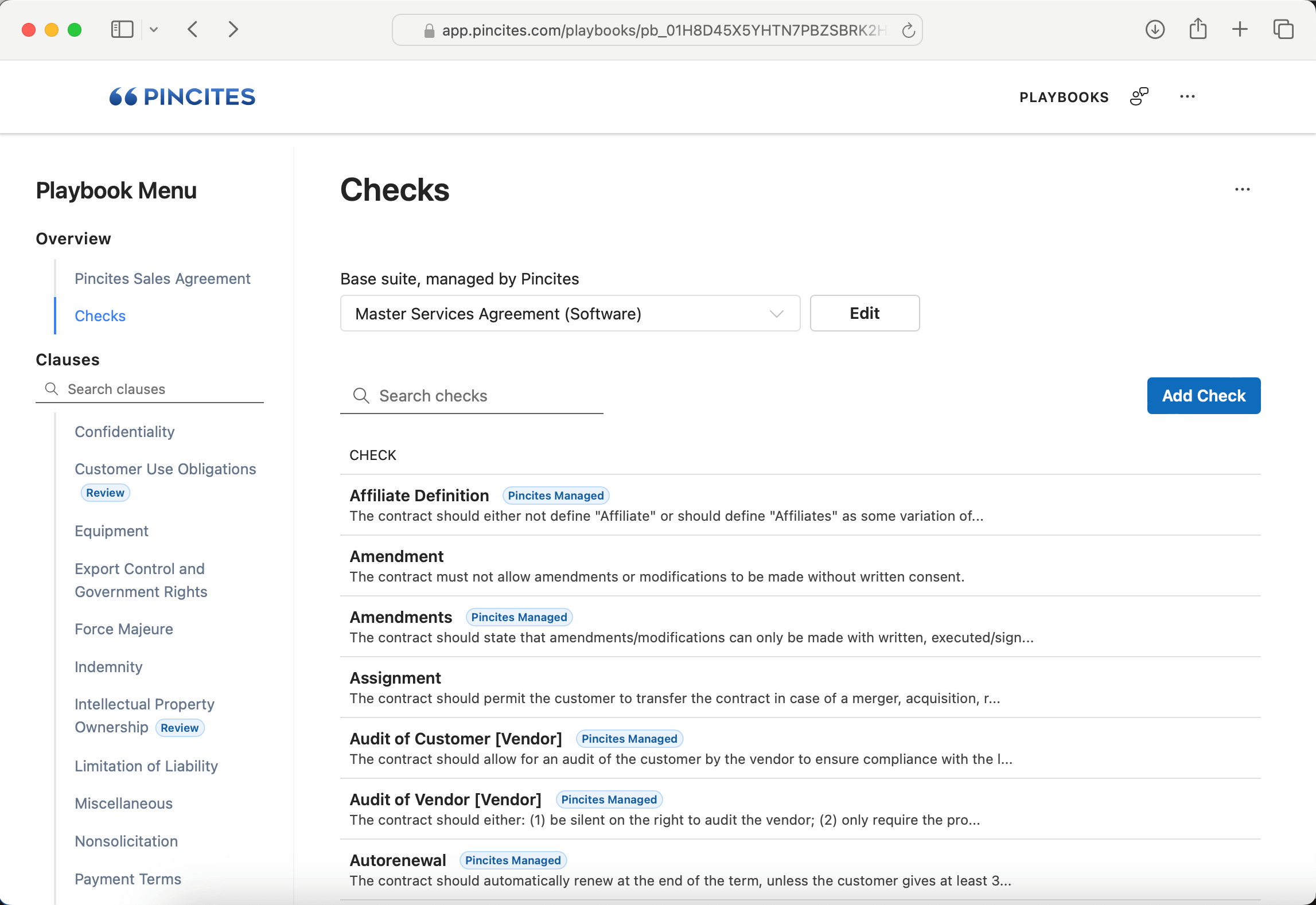Screenshot of a webpage taken from a MacBook, identifiable by the familiar macOS interface. The browser's URL field is centered at the top, displaying the URL: "app.pinsights.com/playbooks/(series of letters and numbers)." 

The webpage itself has a clean, white background. Positioned prominently at the top-left is a logo consisting of two blue quotation marks, followed by the text "PINCITES" in matching blue letters. Adjacent to the logo, on the right, is the word "playbooks" in black font. Nearby, there's an icon consisting of three circles arranged in a triangular formation, complemented by three horizontal dots.

A horizontal gray line runs across the page, providing separation. On the left, there is a vertical menu featuring various navigation options in descending order. The title "playbook menu" is presented in bold, black text at the top. Below this, in smaller text, "overview" is listed. A vertical gray line labeled "pinsights sales agreement" follows.

Blue highlighting indicates the current selection, with the word "checks" written in blue. Below this, a black subheader reads "clauses." A search bar with a white background and gray placeholder text "search clauses" is also evident.

Continuing down the vertical menu, several entries are demarcated by gray lines. These include:

- "confidentiality"
- "customer use obligations"
- A blue button labeled "review"
- "equipment"
- "export control and government rights"
- "force [unreadable word]"
- "indeterminacy"
- "intellectual property ownership"
- Another blue "review" button
- "limitation of liability"
- "miscellaneous"
- "non-solicitation"
- "payment terms"

The layout and interface suggest a professional, document-oriented webpage designed for managing and navigating various legal clauses and agreements.